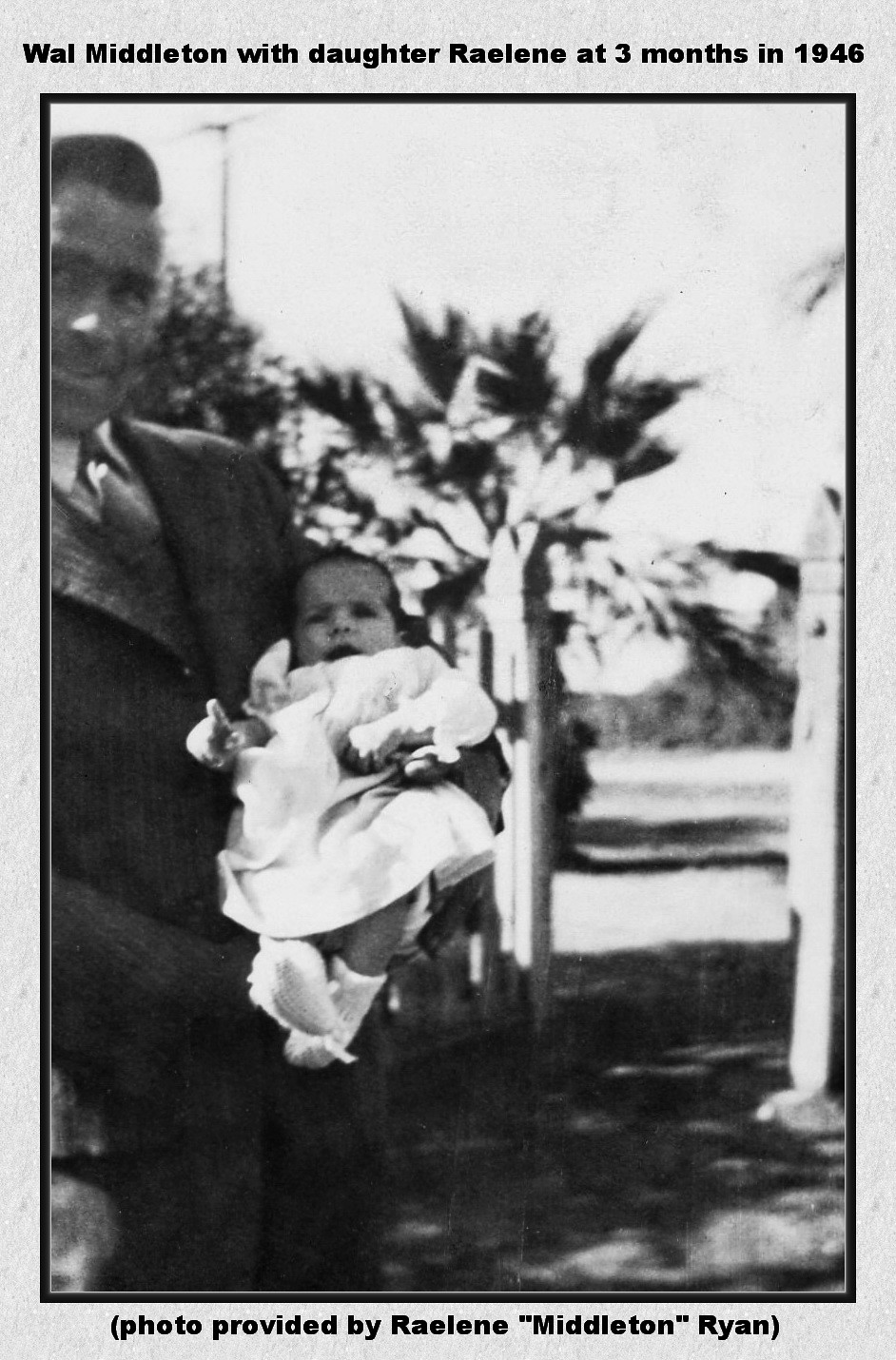This black-and-white photograph, framed by a thick white border, captures a tender moment in 1946 of Wall Middleton with his three-month-old daughter, Raylene. The image, which might have been clipped from a newspaper or a book, is annotated at the top with the caption: "Wall Middleton with daughter Raylene at three months in 1946," and at the bottom it reads, "Photo provided by Raylene Middleton Ryan." Wall, who appears to be in his late twenties or early thirties, is dressed in a dark pinstriped suit with a tie, and his hair is neatly parted to the side. He stands slightly off-center to the left, smiling gently past the camera. Cradled in his arms, baby Raylene wears a delicate white dress and matching booties, with her right hand extended as if pointing. The outdoor setting includes various trees, possibly palm trees, fence posts, a low hill, and an open sky in the background, adding to the nostalgic ambiance of this cherished family photograph.